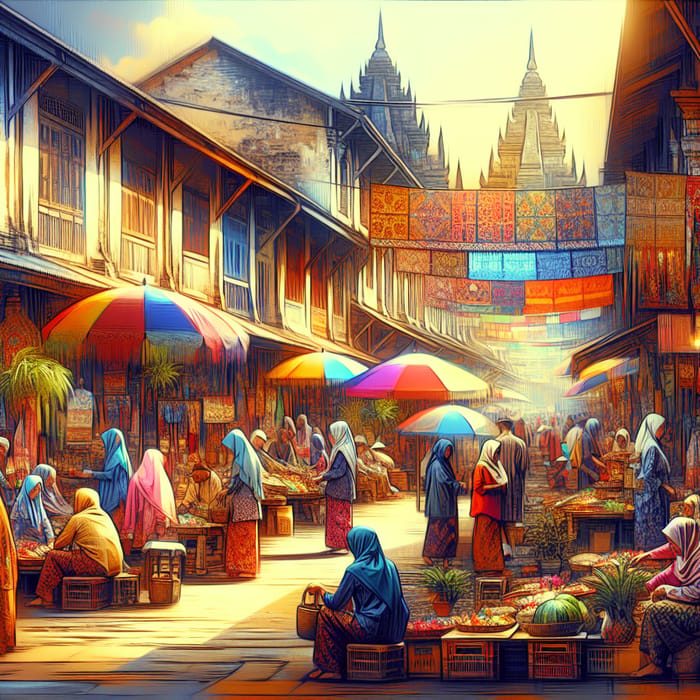This vibrant illustration depicts a bustling marketplace, likely in a Middle Eastern or African setting. The colorful scene features a cobblestone ground bathed in a golden light, indicating early morning or late evening. In the foreground, knee-high tables and crates covered with fruits, including pineapples, line the bottom right corner. Stalls adorned with multi-colored umbrellas stretch along the sides of the roadway, each staffed by modestly-dressed individuals wearing shawls, hijabs, and multicolored clothing in blue, yellow, pink, orange, red, purple, and brown. The people, primarily women, though some men are present, appear faceless yet animated as they engage in shopping and social interactions. Overhead, intricate rugs hang from clotheslines, adding to the market's decor. In the distance, ornate, spiky triangular towers rise above the houses and businesses, further enriching the scene's cultural context.